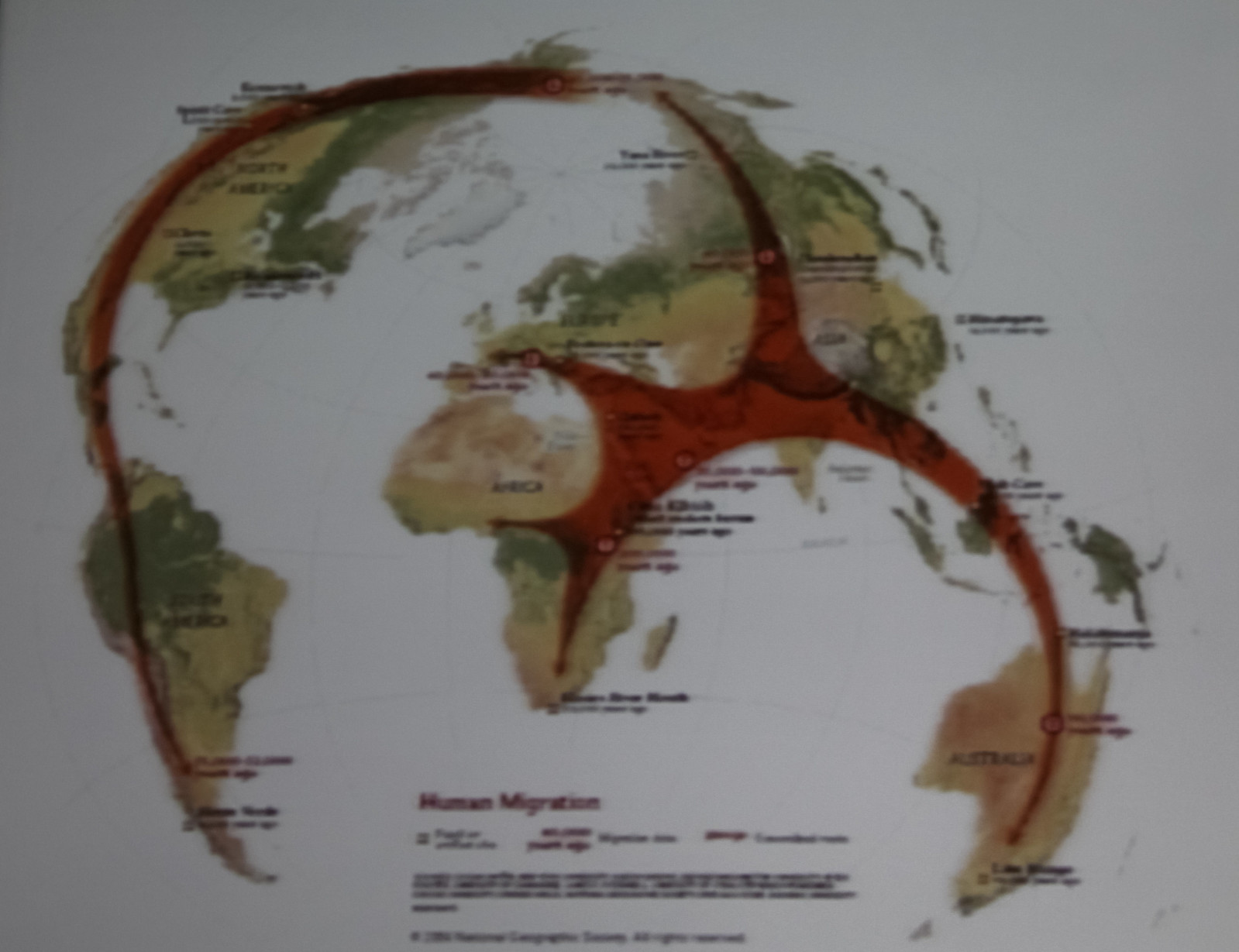This image is a detailed poster of a physical world map showcasing the diverse continents of Earth. The continents—North America, South America, Africa (centered), Europe (above Africa), Asia, and Australia (bottom right)—are illustrated in green and brown hues against a light blue background, representing the ocean. Connecting all these continents are red lines, symbolizing human migration across the globe. Beneath the map, the bold red heading "Human Migration" stands out. Below this heading, there's additional text in black and red, though it is too fuzzy to decipher. At the bottom of the poster, the copyright notice reads, "National Geographic Society, all rights reserved."